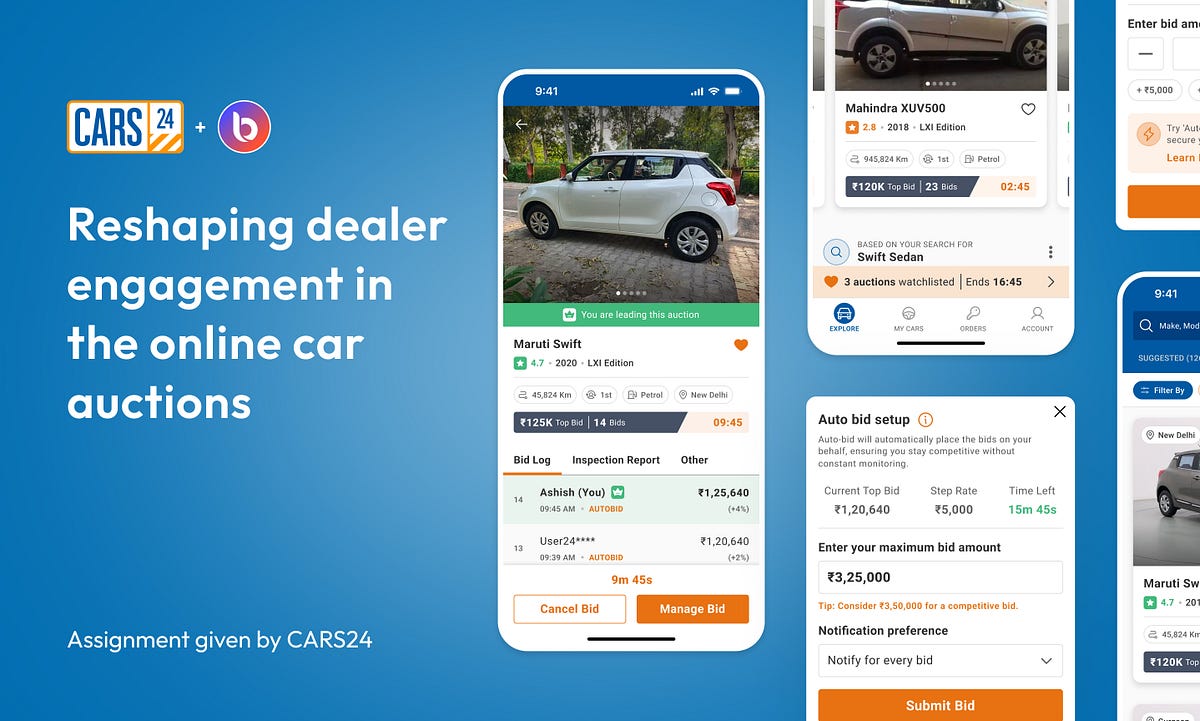A detailed and organized caption for the given image could be:

---

In the image, there is a blue background featuring the Cars24 logo along with a circular icon containing the letter 'B'. The graphic is centered around the theme of reshaping dealer engagement in online car auctions, a concept promoted by Cars24.

Displayed are six screenshots, though only three are fully visible while the others are partially cut off. The first visible screenshot shows a white two-door minivan, identified as a 2020 Maruti LXI edition with a 4.7-star rating. The timestamp on this screenshot reads 9:01 or 9:41. Below the vehicle details, there are options including an orange-underlined "Bid Log", "Inspection Report", and "Other". At the bottom of this section, there are two buttons: a white rectangle labeled "Cancel Bid" and an orange rectangle labeled "Manage Bid".

The second visible screenshot provides details of a Mahindra XUV 500, also rated highly, and displays the Mahindra logo. Beneath this section, there are four icons displayed at the bottom.

---

This caption provides a clear, structured, and detailed description of the elements present in the image.